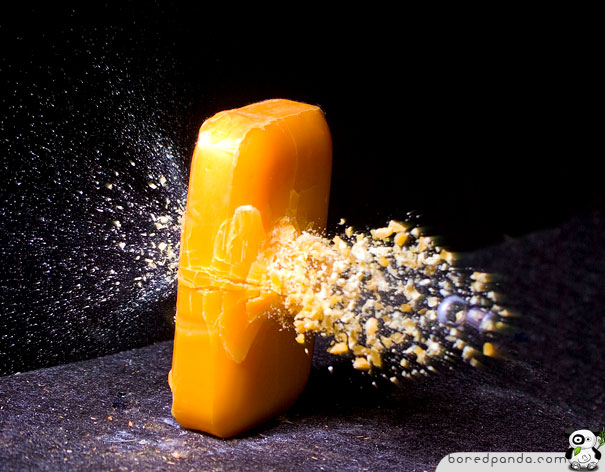This high-speed photograph captures the exact moment a bullet pierces through an orange bar of soap standing upright on a dark surface. The bar of soap, vertically positioned, is centrally illuminated against a solid black background, highlighting its vibrant color. Upon closer inspection, the bullet is seen entering from the left-hand side, where minimal soap fragments are visible, and dramatically exiting through the right-hand side, where an explosion of soap particles and larger chunks burst outward. This dynamic scene is accentuated by the soap cracking in the middle from the bullet’s impact. The surface beneath the soap is dark with a lighter, galaxy-like splatter pattern. The bottom right corner of the image is watermarked with "boredpanda.com" alongside a panda logo, adding a distinct branding element to the composition.